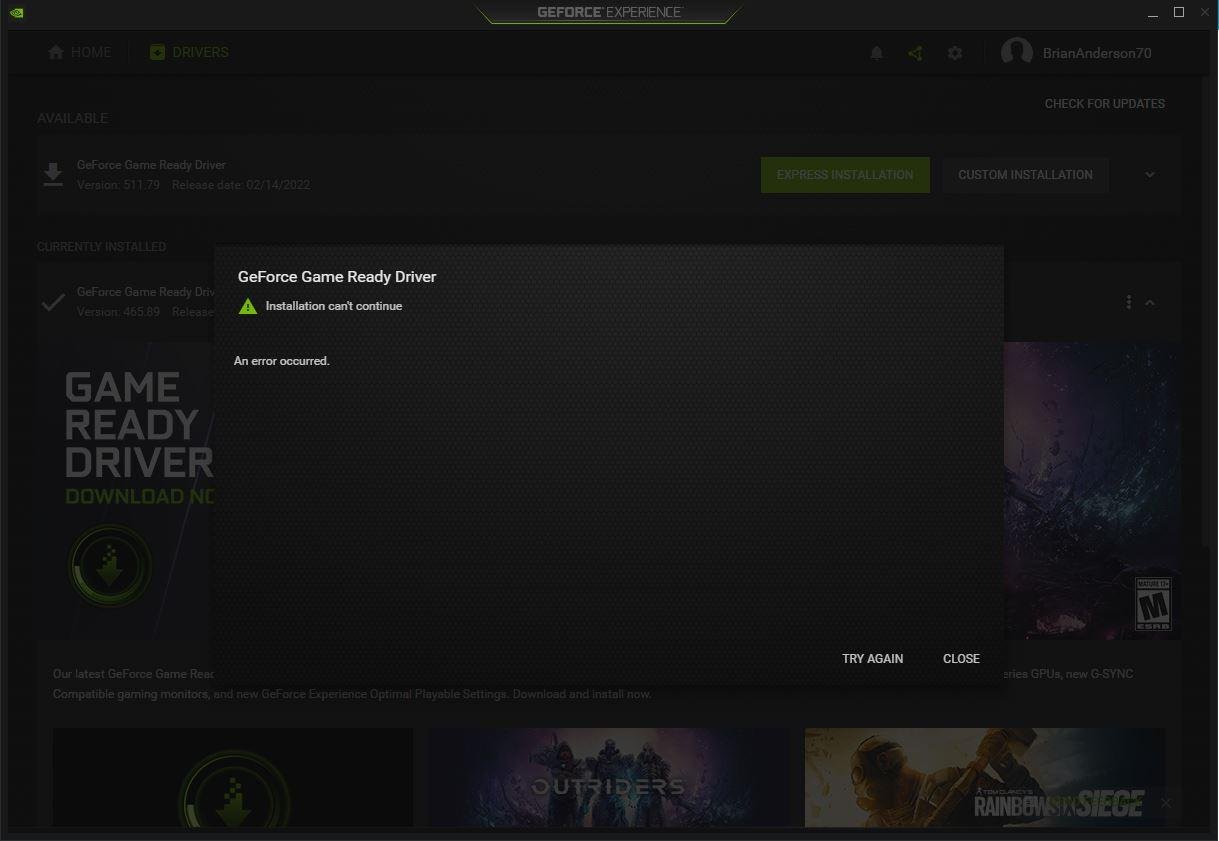A screenshot of the GeForce Experience software is displayed on a computer screen. The application, designed by NVIDIA for managing and updating graphics processing units (GPUs), showcases a sleek user interface dominated by green and black colors. In the background, a series of games, including Outriders and Rainbow Six Siege, are visible, with an M for Mature rating appearing for one of them. Prominent on the screen is a pop-up notification indicating that the "GeForce Game Ready Driver" installation has encountered an error and cannot continue. The user is prompted to "Try Again" or "Close" the message. Additional UI elements are visible in the background, such as options for "Express Installation" and "Custom Installation." The user, identified as Bryan Anderson (70), has signed into the software, and the NVIDIA logo is prominently displayed in the top left corner, signifying the application's origin.